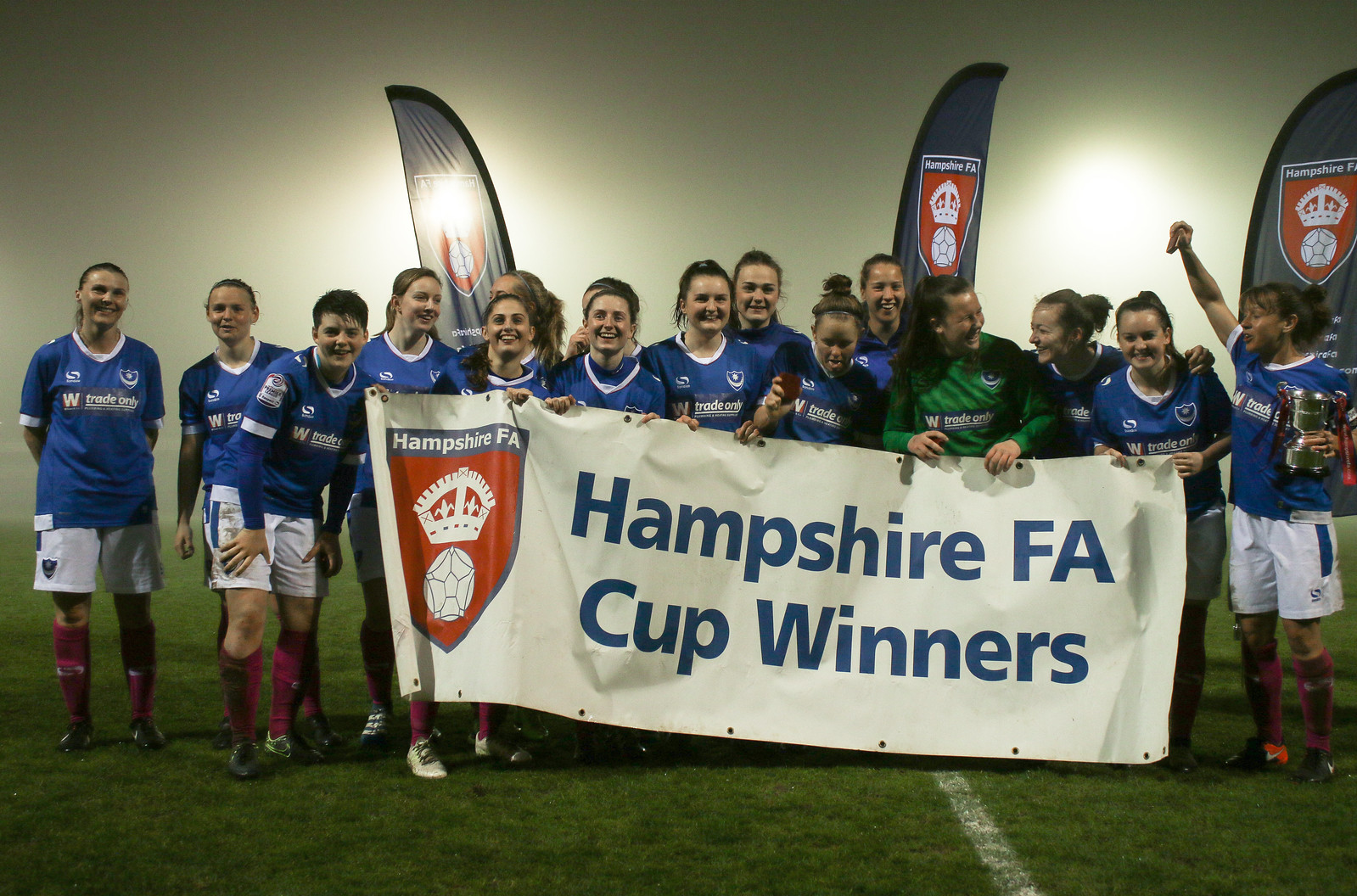The image captures a jubilant women's soccer team, likely composed of around 15 young athletes, gleaming with triumph as they celebrate their victory. They are positioned on a vibrant green field with clear white markings that suggest a goal area. Clad predominantly in blue short-sleeved shirts paired with white shorts and contrasting purple knee-high socks, the focal point of the scene is a large banner they proudly hold in front of them. This banner, white with blue lettering, triumphantly proclaims "Hampshire FA Cup Winners" and features the Hampshire FA emblem—a shield adorned with a crown and soccer ball against a red backdrop. One standout player, possibly the goalkeeper, wears a distinctive green long-sleeved shirt, while another player, beaming with joy, holds up a trophy, her arm raised in celebration. The backdrop behind them is a minimalist whitish-gray, punctuated by several flags that echo the team’s crest, reinforcing their identity and achievement. The team exudes happiness and pride, clearly savoring their hard-won victory.